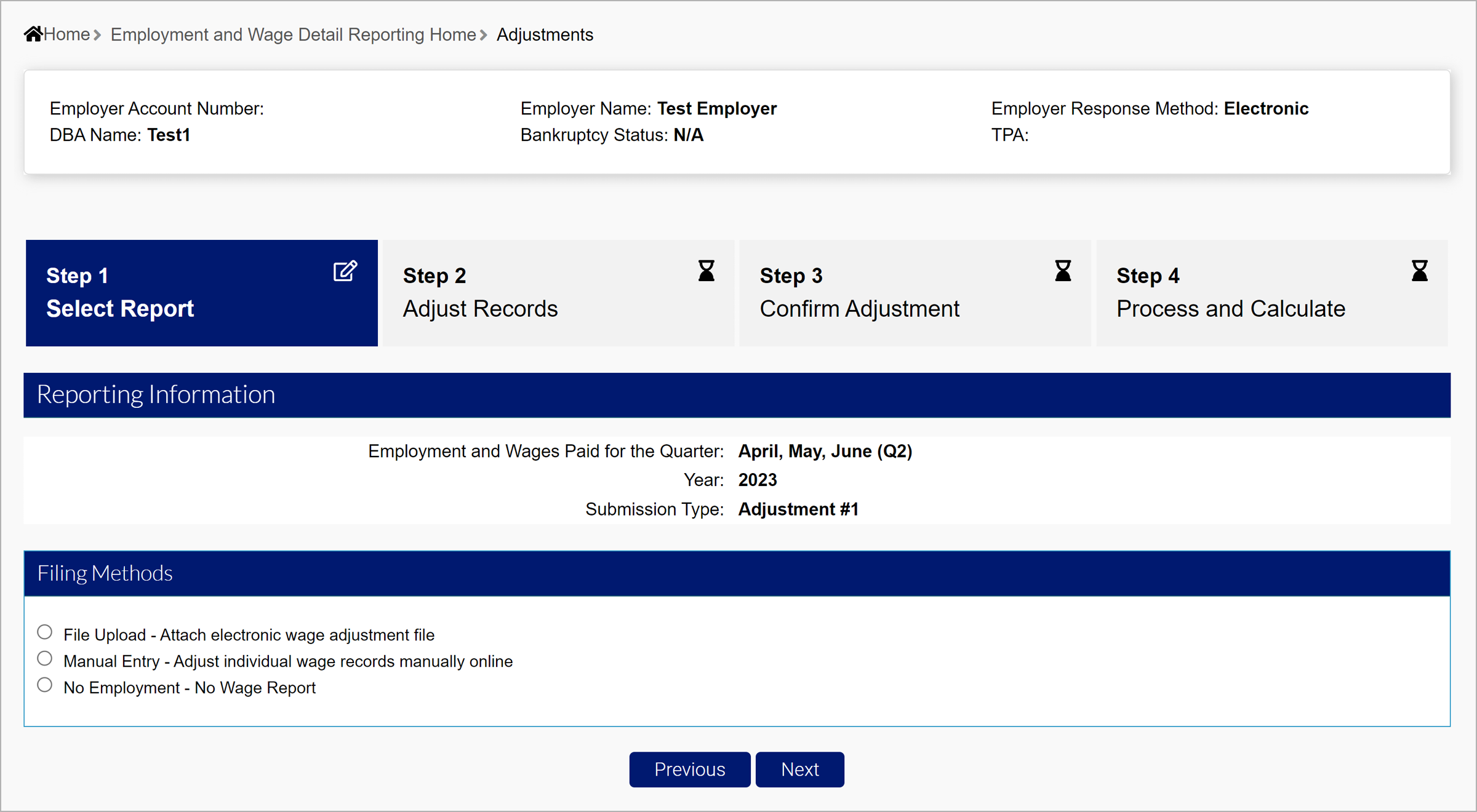A screenshot of an online employment and wage reporting system interface is displayed. In the top-left corner is the home section labeled "Employment and Wage Detail." The main navigation includes tabs such as "Reporting Home," "Adjustments," "Employer Account Number," "DBA and DEM," "Employer Name," and "Test Employee." Key sections titled "Bank Result Status," "Name," and "Employer Response Method" follow, highlighting the method as "Electronic" and related details under "TPA."

The process is broken down into steps:
- Step 1: Select Report (indicated by a blue square).
- Step 2: Adjustment Requirements (with an hourglass icon).
- Step 3: Confirm Adjustment (also with an hourglass icon).
- Step 4: Post and Calculate (again with an hourglass icon).

The "Reporting Information" section displays employment and wages paid for the quarter, specifically mentioning April, May, and June of Quarter 2, Year 2023. The submission type is noted as "Adjustment Number 1."

A blue bar titled "Filing Methods" has various options like File, Apply, Detached, Electronic, Wage Adjust File, Manual Entry, and Adjust Individual Wage Records, with none of them checked. Other functionalities displayed include "No Employment, No Wage Report," with corresponding options for "Previous" and "Next" steps indicated by blue rectangles.

Additional lines and shadows encompass the overall interface layout, adding depth to the visual elements on the screen.